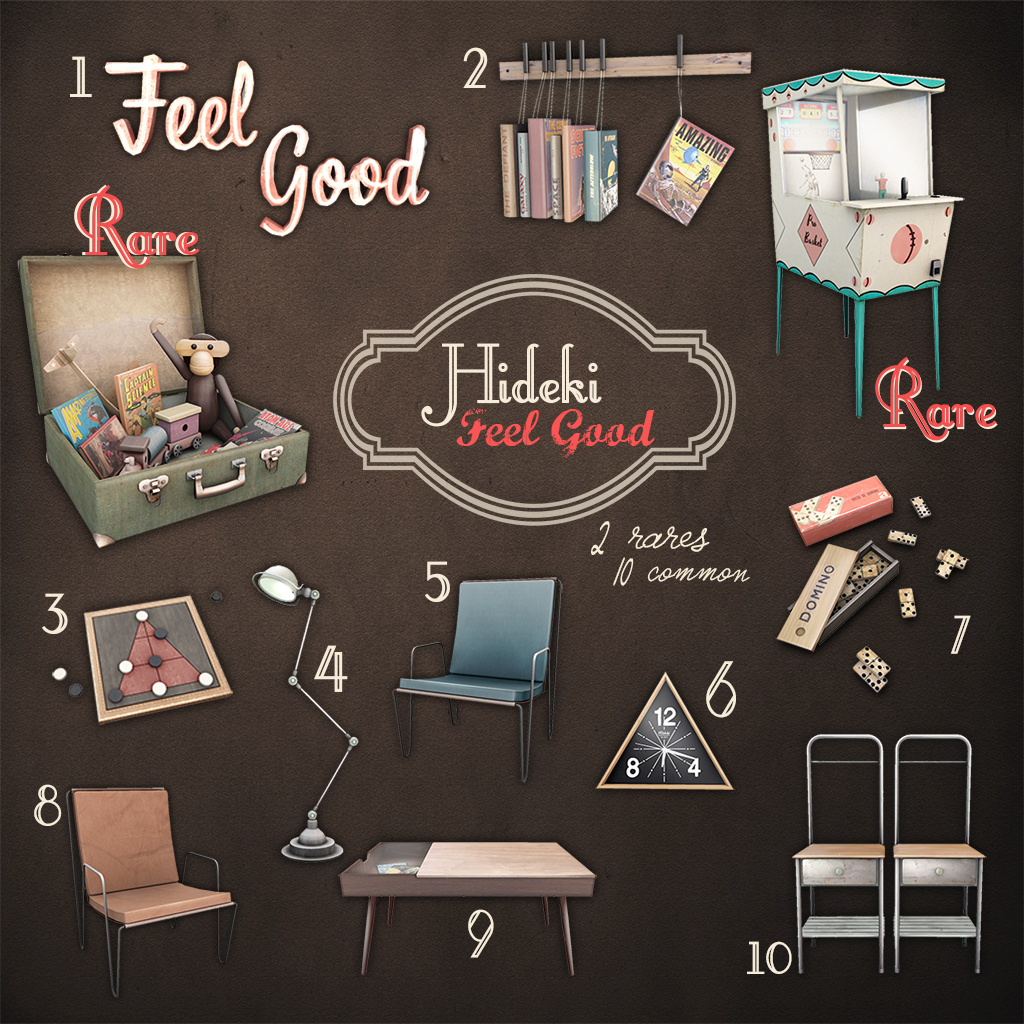The image presents a digital blackboard with a dark backdrop, showcasing various numbered objects, each accompanied by a white numeral from one through ten positioned around the poster. 

In the top center, prominently displayed is a logo reading "Hideaki Feel Good," with "Feel Good" rendered in red ink. Below this central logo are the following items, each indicated by its respective number:

1. The text "Feel Good."
2. A rack attached to a wall with books hanging from it.
3. A game board.
4. A lamp.
5. A chair.
6. A triangular clock.
7. A box of dominoes.
8. A brown chair.
9. A small coffee table.
10. Two aluminum chairs.

Additionally, the poster features the text "Rare," indicating that some objects, like an arcade machine and a box of toys, are special prizes, with two being classified as rare and ten as common. The image evokes a collage-like style with a diverse palette, including black, white, pink, red, purple, yellow, light blue, maroon, and gray.